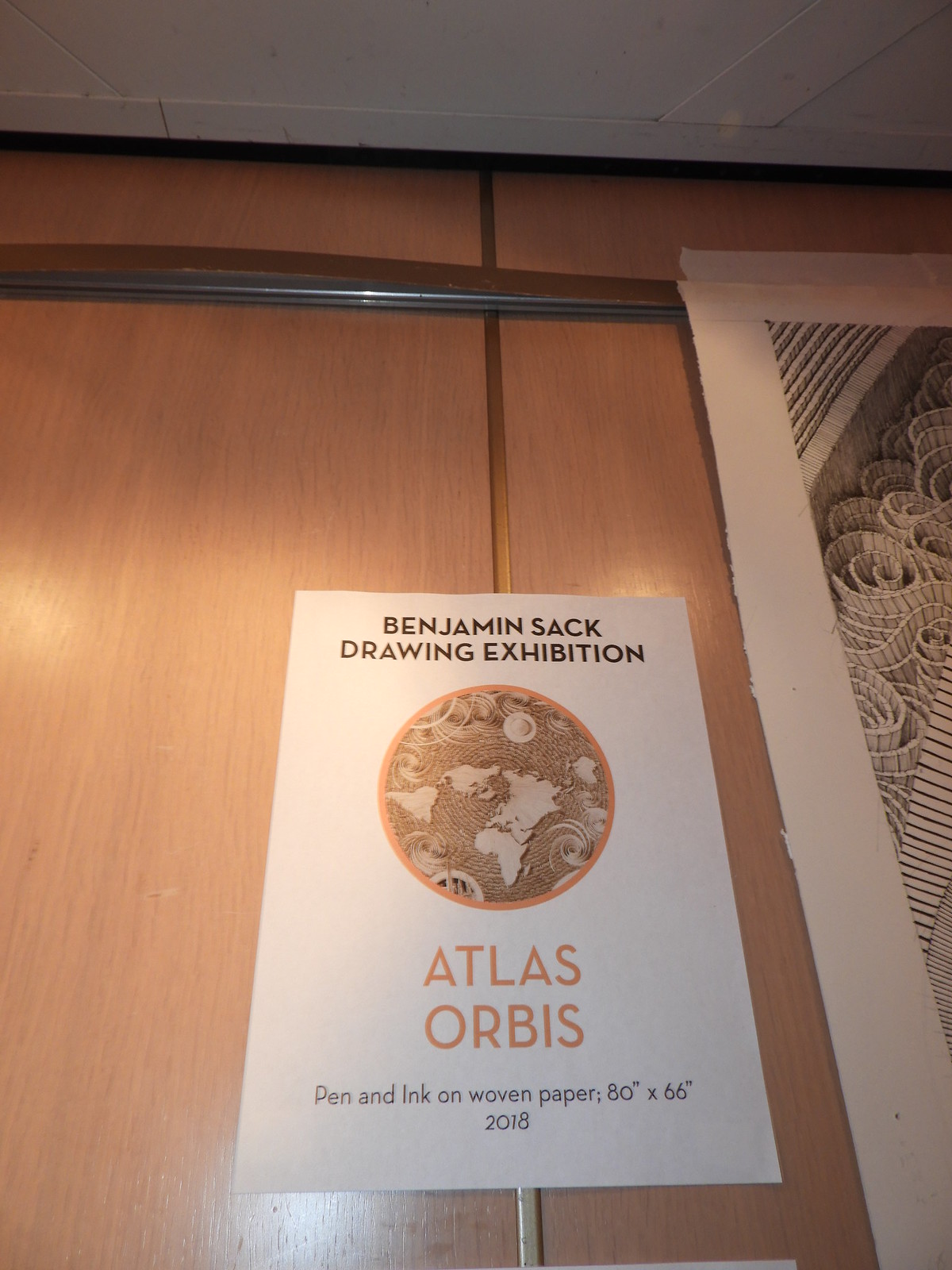The image depicts a white paper sign attached to a light oak-colored wooden wall, which features the detail of a gold or silver stripe giving it a distinct separation. The sign is a vertically-oriented rectangle. At the top of the sign, bold black text announces "Benjamin Sack Drawing Exhibition." Below this, in beige or orange font, reads "Atlas Orbis." Centrally positioned on the sign is a circular image, depicting a detailed pen and ink drawing on woven paper that resembles a map of the world with numerous intricate swirls. This central piece provides a preview of the artwork on display. Below the circular image, in dark writing, it states "Pen and Ink on Woven Paper, 80 inches by 66 inches, 2018." Adjacent to the sign, we can see the edge of another white poster, possibly part of the same exhibition.